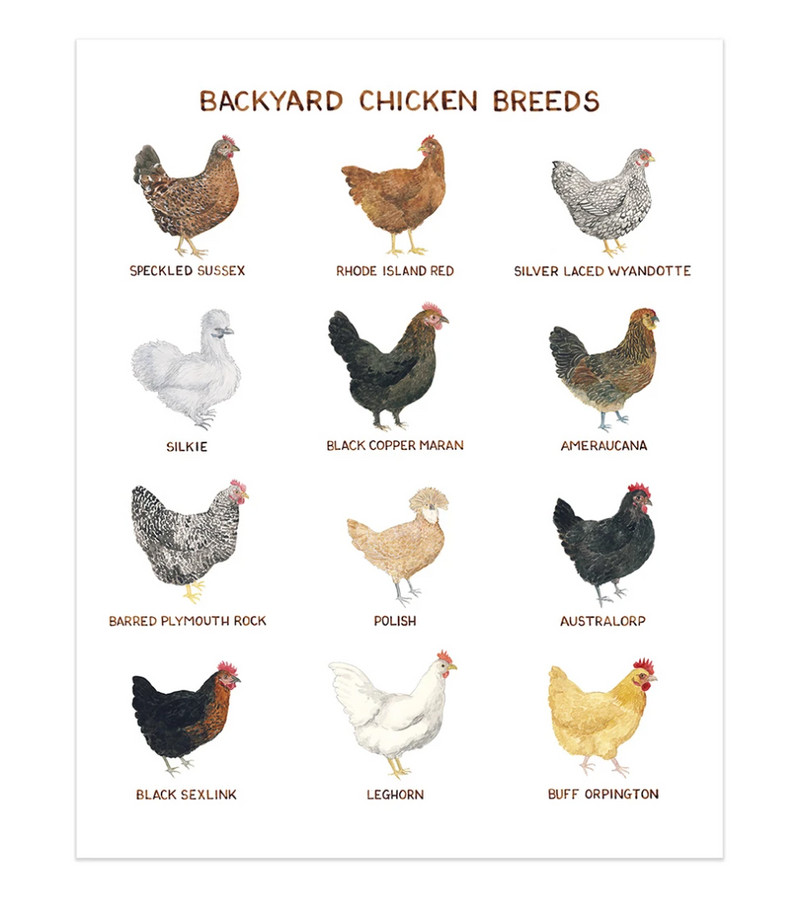The image is a detailed poster titled "BACKYARD CHICKEN BREEDS" in brown capital letters at the top, set against a solid white background. Organized into four rows, each containing three chickens, the chart showcases a total of 12 different chicken breeds, each vividly illustrated from a side view with a brown text label indicating the breed. Starting from the top left and moving left to right, the breeds are listed as follows: Speckled Sussex (a brown chicken with white and gray spots), Rhode Island Red (a brown chicken), Silver-Laced Wyandotte (a white chicken with black lines and spots), Silky (a puffy, fuzzy-looking white chicken), Black Copper Maran (a black chicken), Americana, Barred Plymouth Rock, Polish, Australorp, Black Sexlink, Leghorn, and Buff Orpington. Each chicken features distinctive colors and patterns, along with the characteristic red comb on top of its head, providing a comprehensive visual guide to different backyard chicken breeds.